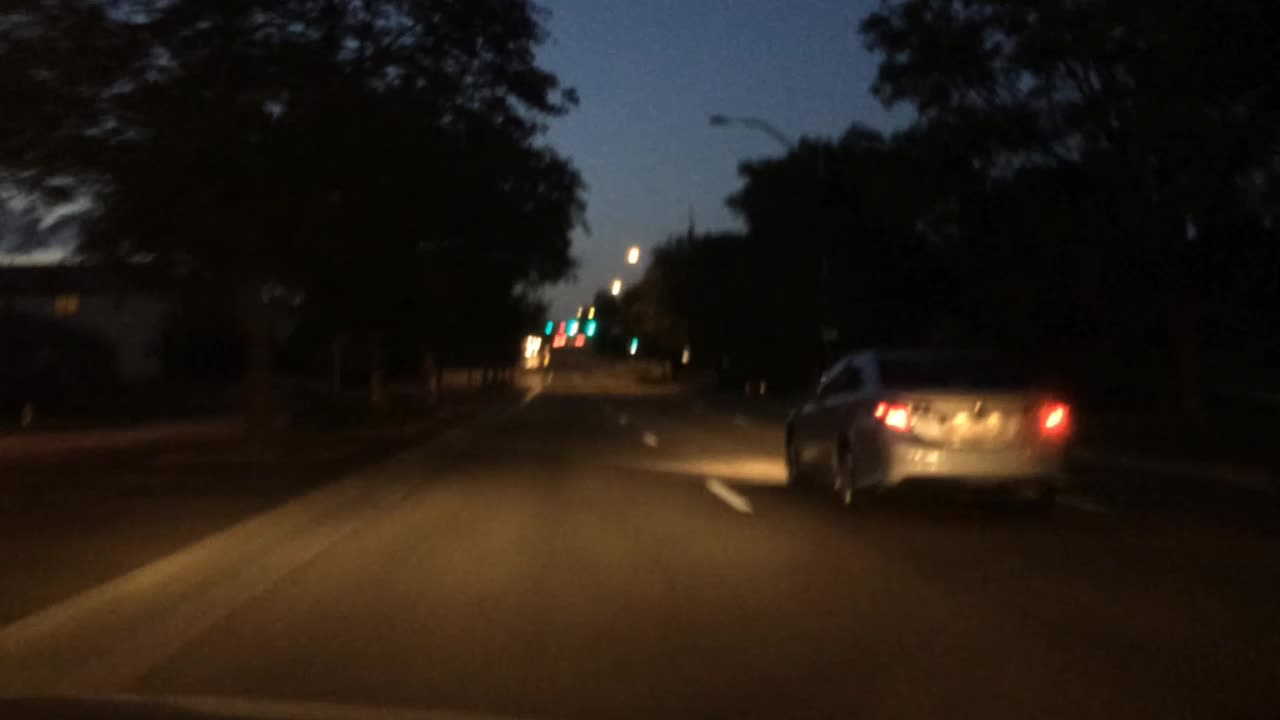The nighttime photograph captures a view from the left lane of a three-lane road, suggesting it may be a residential street rather than a freeway. The scene is quite dark, indicative of dusk just as nightfall is approaching. Silhouetted trees flank both sides of the road, and a non-operational streetlight is visible about 20 car lengths ahead on the right. Another car, a light-colored or silver sedan, occupies the middle lane and is about two car lengths in front of the photographer, with its brake lights illuminated. The scene also features distant streetlights and intersection signals—green, red, and blue—blurring into the background. A sparsely lit window hints at a house presence amid the large trees.